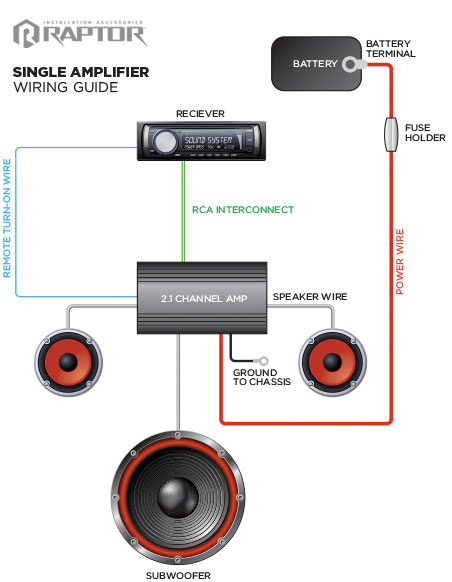This detailed illustration on a white background, titled "Raptor Single Amplifier Wiring Guide," meticulously depicts the intricate electronic wiring setup for a sound system. In the upper left corner, a symbolic letter "R" is set against a hexagon, both in gray, accompanied by the word "Raptor" and some unreadable smaller text. Below these symbols, the title "Single Amplifier" is prominently displayed in bold text, followed by the label "Wiring Guide" in black.

The diagram features various key components, including a black rectangular receiver with a white circle, a black 21-channel amplifier labeled in white text, and a gray subwoofer adorned with a red circle. Two wires emerge from the amplifier: a green RCA interconnect line extending downward from the receiver and a blue remote turn-on wire branching left, then downward, then right.

The 21-channel amplifier is connected to two speakers, one on each side. Additionally, it has a line extending to a subwoofer below it. A red power wire extends to the right and upward, connecting to the battery terminal in the upper right corner, with a fuse holder affixed to this power wire. The diagram efficiently visualizes the entire wiring setup, with colored arrows and lines indicating connections, providing a comprehensive guide for setting up the speaker system.